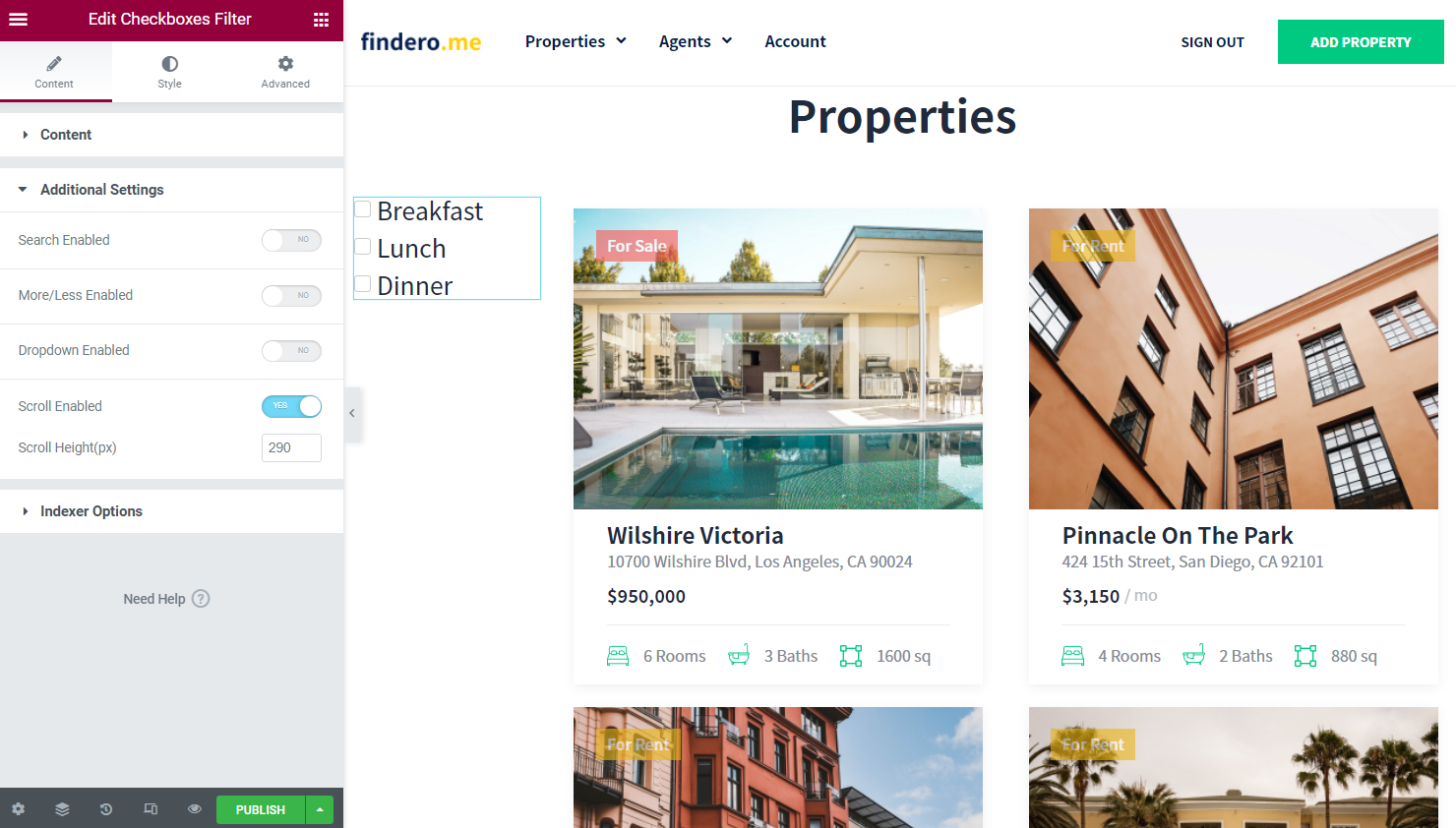**Detailed Caption:**

This is a web page showcasing various properties, displayed against a white background. On the very left side, approximately a quarter way from the left edge, there is a dark red banner featuring a vertical stack of three white lines resembling a menu symbol. In the center of this banner, the text "Edit Checkboxes Filter" appears in white. To the right of this text, another similar menu symbol is visible.

Below this, three tabs are present: the first tab labeled "Content" is underlined in red, the second tab labeled "Style" sits in the middle, and the third tab labeled "Advanced" on the right, is marked with a small cog symbol indicating settings options. Directly beneath these tabs, the word "Content" reappears with a light blue or gray horizontal line below it.

Further down, the section titled "Additional Settings" features interactive toggle buttons aligned to the right of each setting that can be switched to "Yes" or "No." Near the bottom of the section, a large light blue or gray square centered towards the top displays the text "Need Help" accompanied by a question mark icon. Below this, various symbols are arranged in a row.

At the bottom right corner of the page, a green rectangle contains the text "Publish." Located near the top of the page, "Finder.me" is displayed, providing site information. Underneath this title in the center of the page, the word "Properties" appears in black.

On the left, below the "Properties" heading, there is a vertical list with "Breakfast, Lunch, and Dinner," accompanied by checkboxes for selecting options. 

The page showcases four different properties: the first two properties are displayed in the middle section with comprehensive details shown to the right of each. The latter two properties are presented below; however, only partial views of these properties are visible, without additional information.